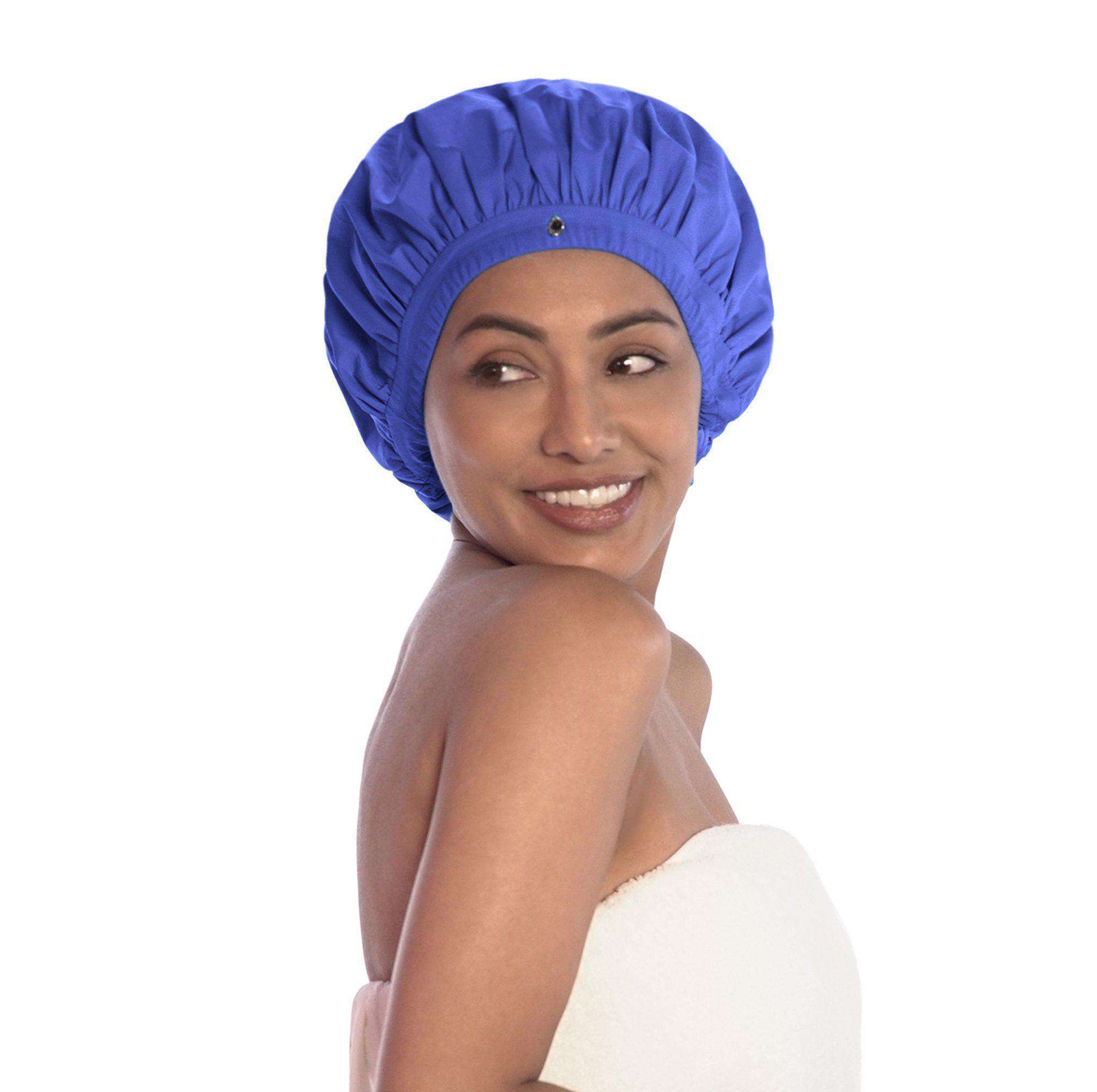The image features a middle-aged woman with tan skin and brown eyes, wrapped in a white towel that covers her from just below her neck to her upper waist. She has a deep blue shower cap on her head, which completely hides her hair. Her body is turned to the right side of the picture while she gazes over her right shoulder with a wide, engaging smile. Her right arm hangs naturally by her side. The backdrop is neutral, which makes the blue of the shower cap stand out prominently. The woman’s beautiful features are highlighted by her wide eyes, well-shaped eyebrows, and radiant smile, possibly suggesting that the shower cap might be the focus of the image.